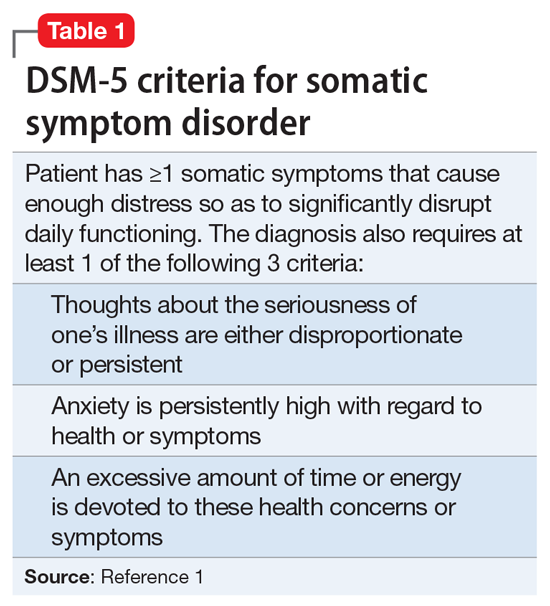This image depicts a section of a website dedicated to medical information. At the top of the image, there is a label "Table 1" displayed in white font within a red circular background. A line extends from this circle to the left and then descends vertically, forming a partial outline around the corner of the webpage.

The primary content of the image centers around the DSM-5 criteria for diagnosing somatic symptom disorder. The text specifies that a patient must exhibit one or more somatic symptoms that cause enough distress to significantly disrupt daily life. In addition, the diagnosis requires at least one of the following three criteria:
1. Disproportionate or persistent thoughts about the seriousness of one's illnesses.
2. Persistent high levels of anxiety concerning health or symptoms.
3. An excessive amount of time or energy focused on health concerns or symptoms.

The information is organized in a visually structured manner with alternating light blue and darker blue boxes. Below this table, the word "Source" appears in bold black letters, followed by a semicolon and a reference marked with the number one.

Aside from the red circular background and blue-colored boxes, the overall color scheme of the webpage is primarily white, providing a clean and minimalistic look.